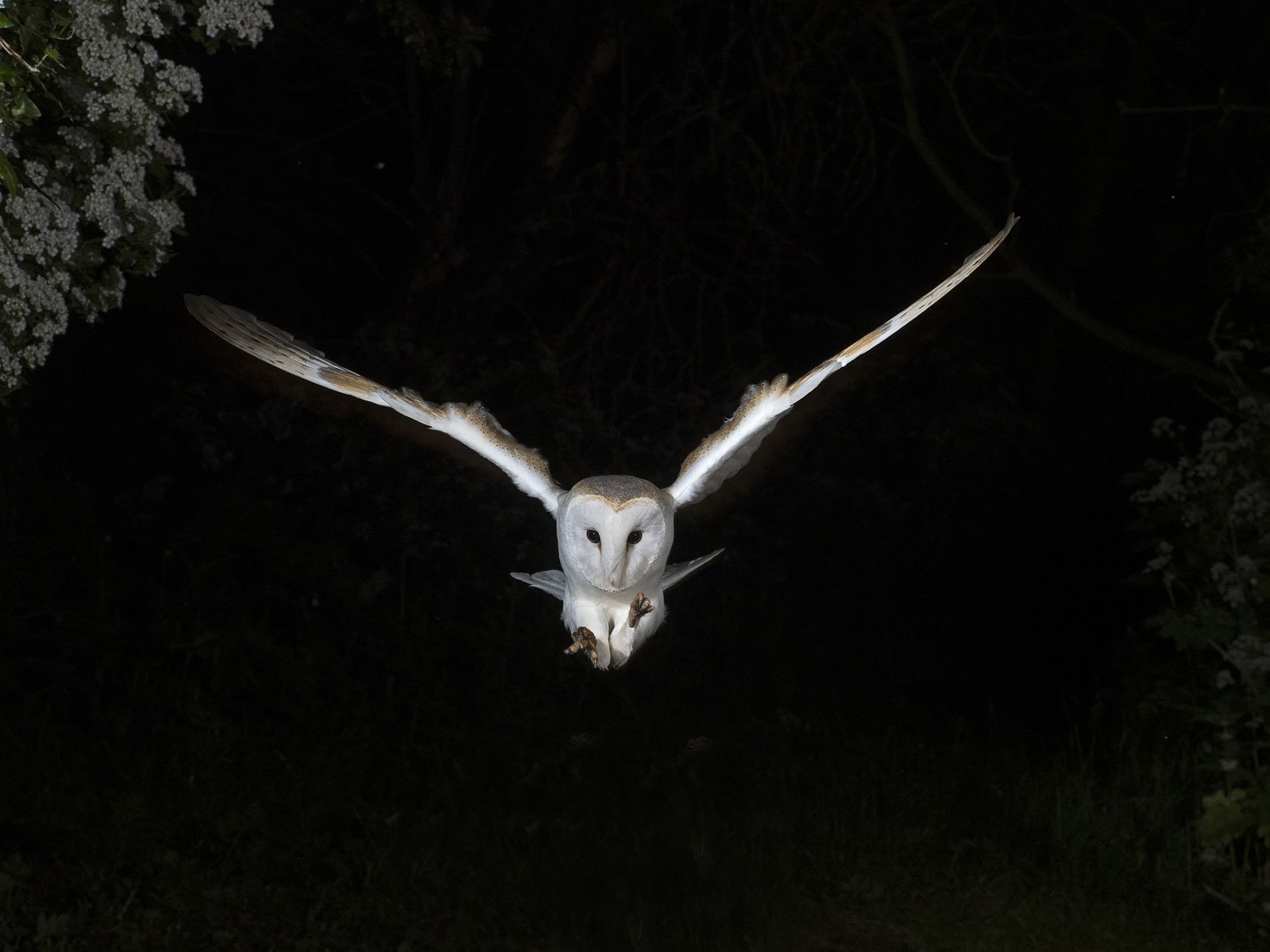In the center of this striking nighttime image, a white-faced owl with a darker gray head dominates against a completely black background. The highly detailed photograph captures the owl mid-flight, wings spread wide in a dramatic and dynamic pose. Its long wings, which are dark gray on the outside and white on the inside, give the impression of immense power and readiness. The owl's intense, forward-facing gaze and outstretched claws suggest it is about to make a landing or seize prey. The scene is nuanced with small, but telling details: a thin, mesh-like object appears to hang from the owl's beak, and the upper left corner features faintly illuminated leaves, likely part of a tree. Similarly, a barely visible plant occupies the bottom right corner, adding depth and context to the otherwise stark and haunting tableau. The entire composition conveys a palpable sense of anticipation and the quiet ferocity of a nocturnal hunt.